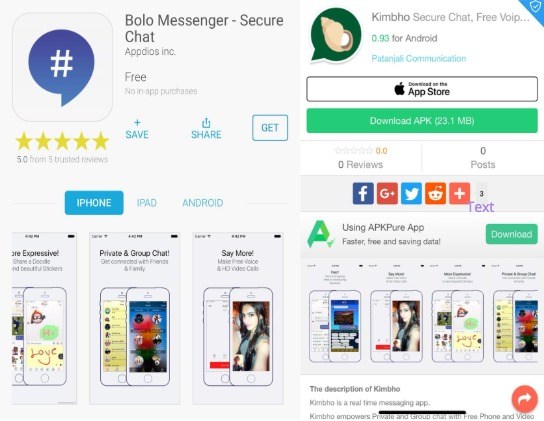The image consists of two side-by-side screenshots featuring advertisements for secure chat applications. 

On the left, the advertisement for "Bolo Messenger" exhibits a visually appealing design with a predominant color scheme of blues, yellows, and blacks. At the bottom of this section, there are images of three iPhones showcasing various features of the Bolo Messenger app.

On the right, the advertisement for "Kimho Secure Chat" is also highlighted. This section features four iPhones at the bottom, presenting different facets of the Kimho Secure Chat app.

The background of the combined image is uniform white, making it challenging to differentiate where one advertisement ends and the other begins. Both ads appear to promote their respective apps' availability on the App Store. The overall layout creates a colorful and vibrant visual experience.